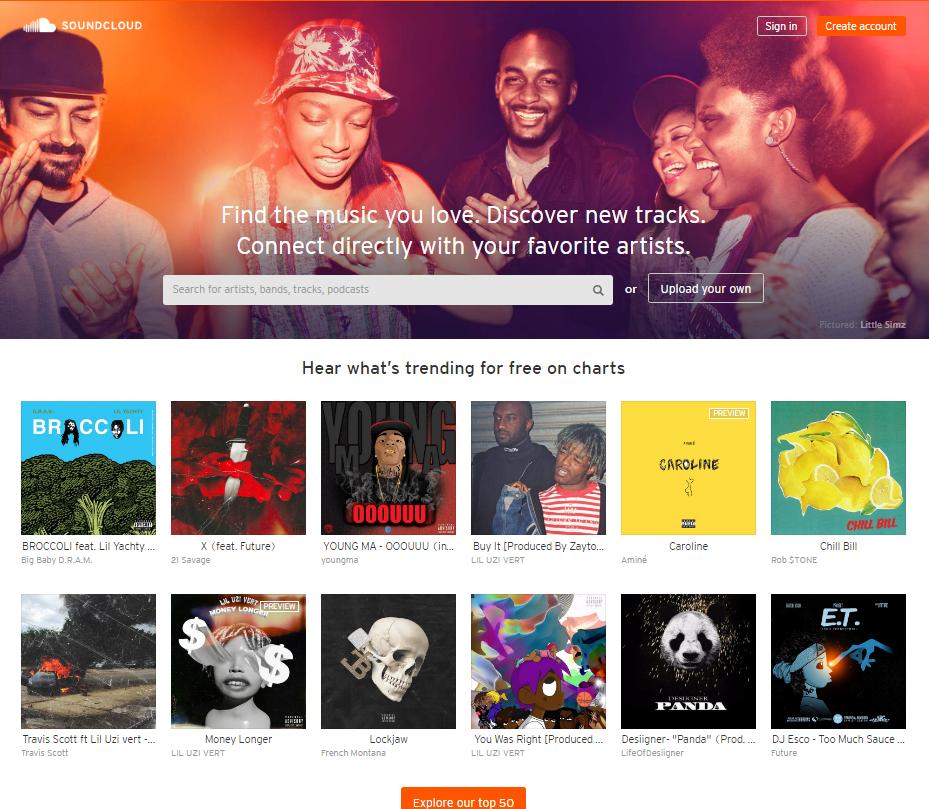The image is a detailed screenshot of the SoundCloud website interface. In the top left corner, the iconic SoundCloud logo, resembling a cloud, is prominently displayed next to the site's name, 'SoundCloud.' On the top right, users can spot the 'Sign In' button alongside a 'Create Account' button, the latter featuring an eye-catching orange rectangle background.

Dominating the top section of the website is a compelling tagline that reads, "Find the music you love. Discover new tracks. Connect directly with your favorite artists." Below this, a sizable search bar invites users to "Search for artists, bands, tracks, and podcasts," with an additional option to "Upload your own." The "Upload your own" text is embedded in a clickable white rectangle.

The background of this upper segment is lively, depicting a photograph of six spirited people who appear to be dancing and reveling in music, smiles lighting up their faces.

Further down, the page encourages users to "Hear what's trending for free on charts," listing the top trending tracks. This section is organized into two rows, each containing six songs, accompanied by their respective album artwork. At the very bottom center of the page, there is an 'Explore our Top 50' button, also emphasized in an orange rectangle.

The charts feature popular tracks including:
- "Broccoli" featuring Lil Yachty,
- "X" featuring Future,
- "OOOUUU" by Young M.A.,
- "Buy It" by Lil Uzi Vert,
- "Caroline" by Aminé,
- "Chill Bill" by Rob $tone featuring J. Davi$ & Spooks.

The second row highlights:
- "goosebumps" by Travis Scott featuring Kendrick Lamar,
- "Money Longer" by Lil Uzi Vert,
- "Lockjaw" by French Montana featuring Kodak Black,
- "You Was Right" by Lil Uzi Vert,
- "Panda" by Desiigner,
- "Too Much Sauce" by DJ Esco featuring Future & Lil Uzi Vert.

Each song is complemented by its album art, creating an engaging visual experience for the user.